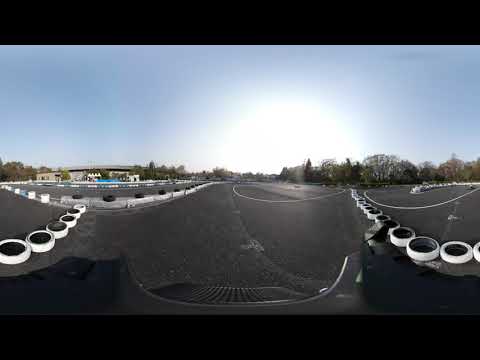The image is a panoramic photograph depicting a racetrack. The central focus is the dark black track itself, bordered by white tires with black centers laid flat along both sides, guiding the path. The pavement of the track is a prominent gray tone. In the distance on the right side of the image, there is a flat-roofed building flanked by trees, complemented by additional trees further back. The left side of the image also features trees in the background, with buildings visible further off. The sky, which occupies a significant portion of the image, is a clear light blue, with the sun's bright aura visible near the middle center, casting a natural glow over the scene. The overall composition shows a detailed mix of elements including the tires that define the edges, the angular views of the track, and the scenic natural and architectural backdrop, all harmonized under a bright, sunlit sky.